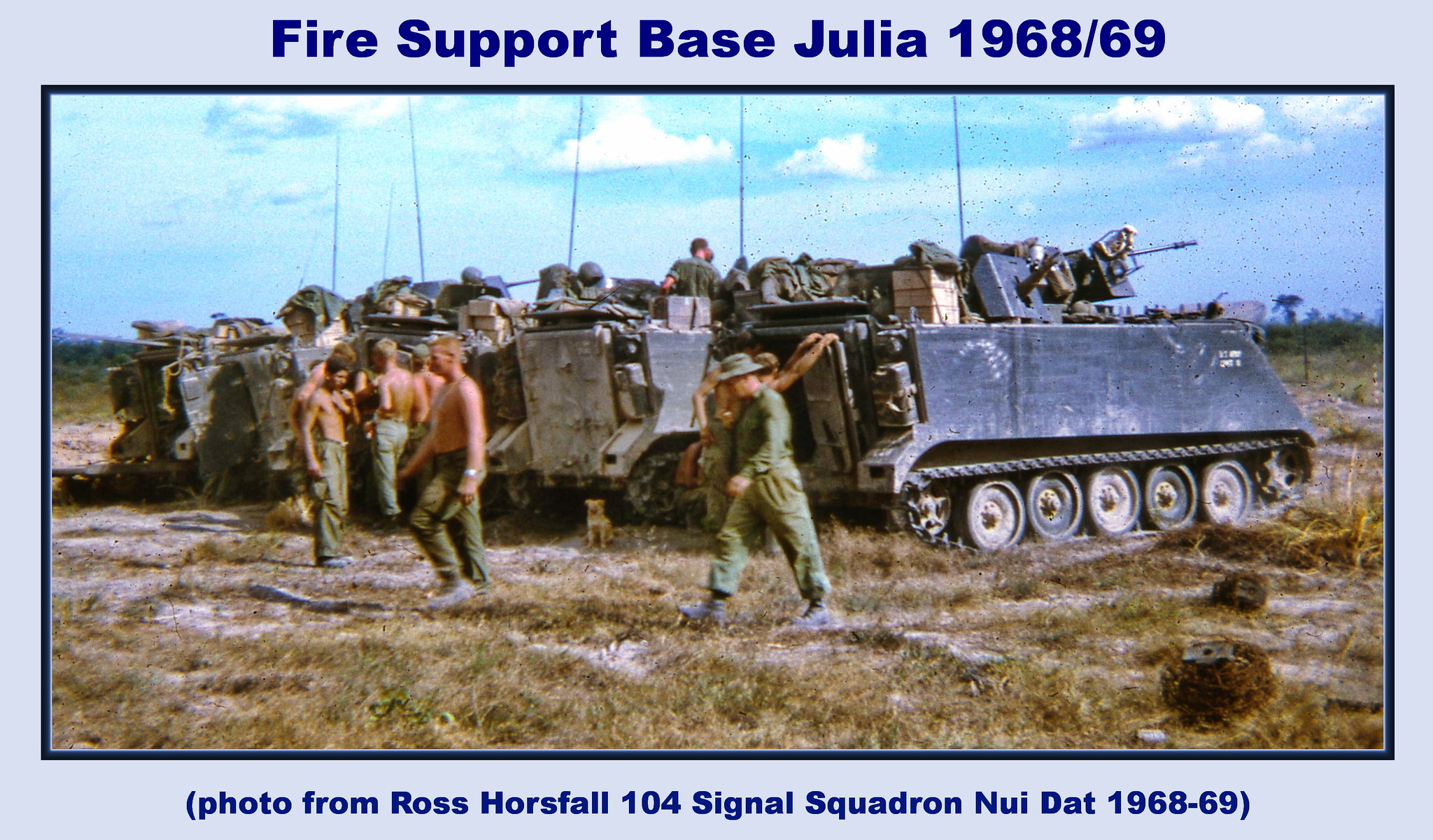The image shows a grainy, sepia-toned photograph capturing a moment from the Vietnam War at Fire Support Base Julia between 1968-1969. In the foreground, there are several soldiers, most of them shirtless, some dressed in pants, and a few wearing shirts, walking around or sitting behind a line of tanks. The tanks, estimated to be four to six in number, are positioned with their guns facing to the right. The scene is set against a backdrop of sparse, dead grass through which the bare ground is visible. A dog sits calmly in the middle of this array. Above the tanks, the sky is blue with white clouds, contributing to the faded, nostalgic tone of the photograph. Notably, the image is bordered in blue, with text at the top stating, "Fire Support Base Julia, 1968-69," and at the bottom, attributing the photo to Ross Horseville (often transcribed as Horse Fall), from the 104 Signal Squadron at Nui Dat, 1968-69.